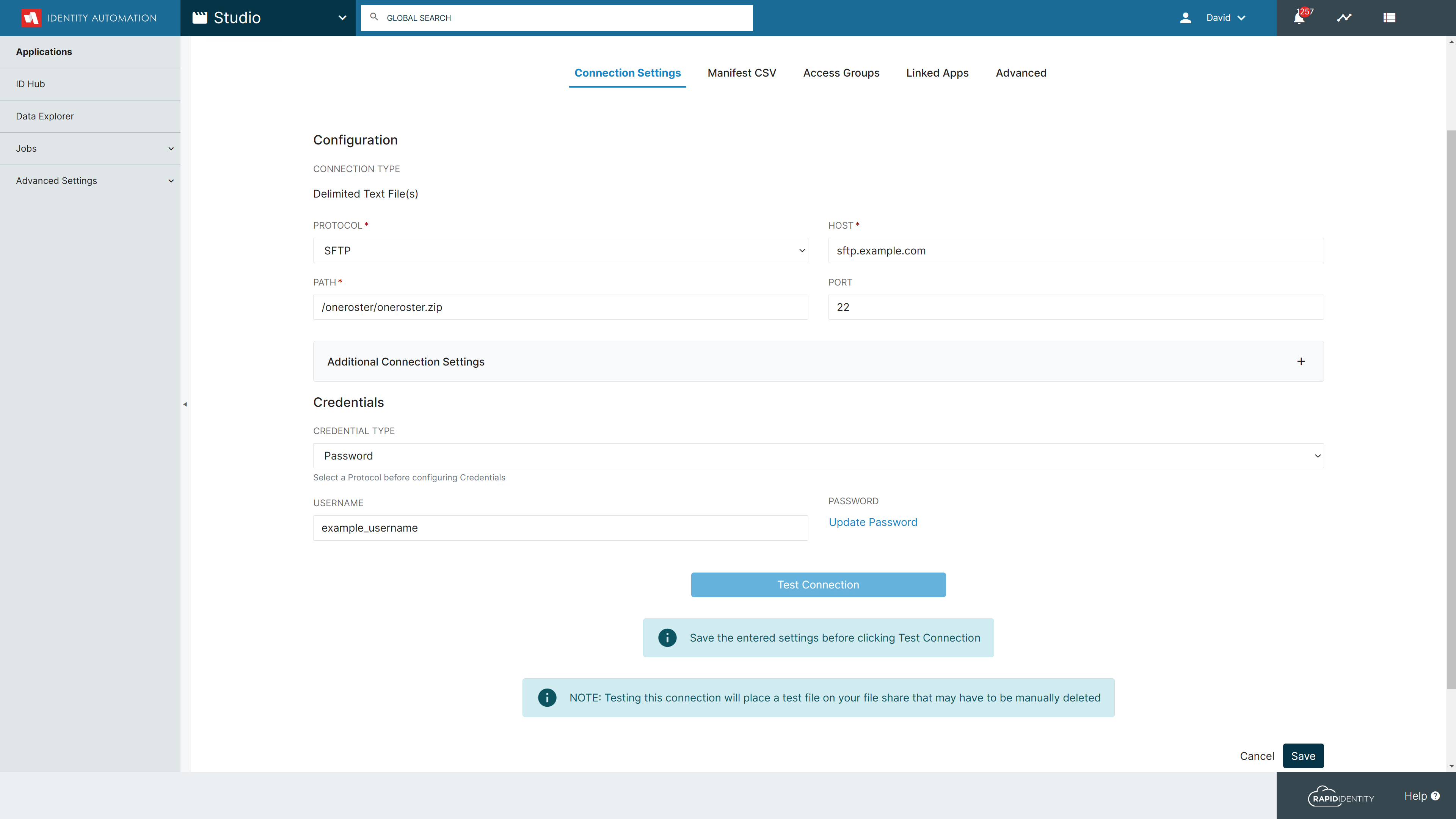The image showcases a detailed user interface within an application called "Identity Animation Studio." In the top left corner, the title "Identity Animation" is prominently displayed on a white background. Below this, a global search bar is visible, followed by sections labeled "David" and "Bell," with a total of 5 items listed.

On the right side, there is a large column that organizes various sections, which include "Applications," "IO Hub," "Data Explorer," "Jobs," and "Advanced Settings." Below these sections, there is a subset titled "Connection Settings," which encompasses several configuration options such as "Manifest CSV," "Access Groups," "Link Tabs," "Advanced Configuration," and more.

Details under the "Connection Settings" include:
- Connection type: Delimited text files
- Protocol: SFTP
- Path: one roster/one roster.zip
- Host: sftp.zip.com
- Port: 22
- Additional connection settings, including credentials where users need to input a username (example_username) and password (password).

Important instruction text is displayed, suggesting users must select a protocol before configuring credentials. There is also a blue bar containing options for "Test Connection" and a reminder to save settings before testing. Notices warn that testing is scheduled and that users should ensure files are shared correctly as they might be deleted otherwise. The bottom right corner features options for "Cancel" and "Save."

Additionally, the interface displays a service name, "Rapid Identity," next to a "Help" button with a scroll bar on the side. The atmosphere of the interface suggests it is a productive and organized morning within this workflow environment.